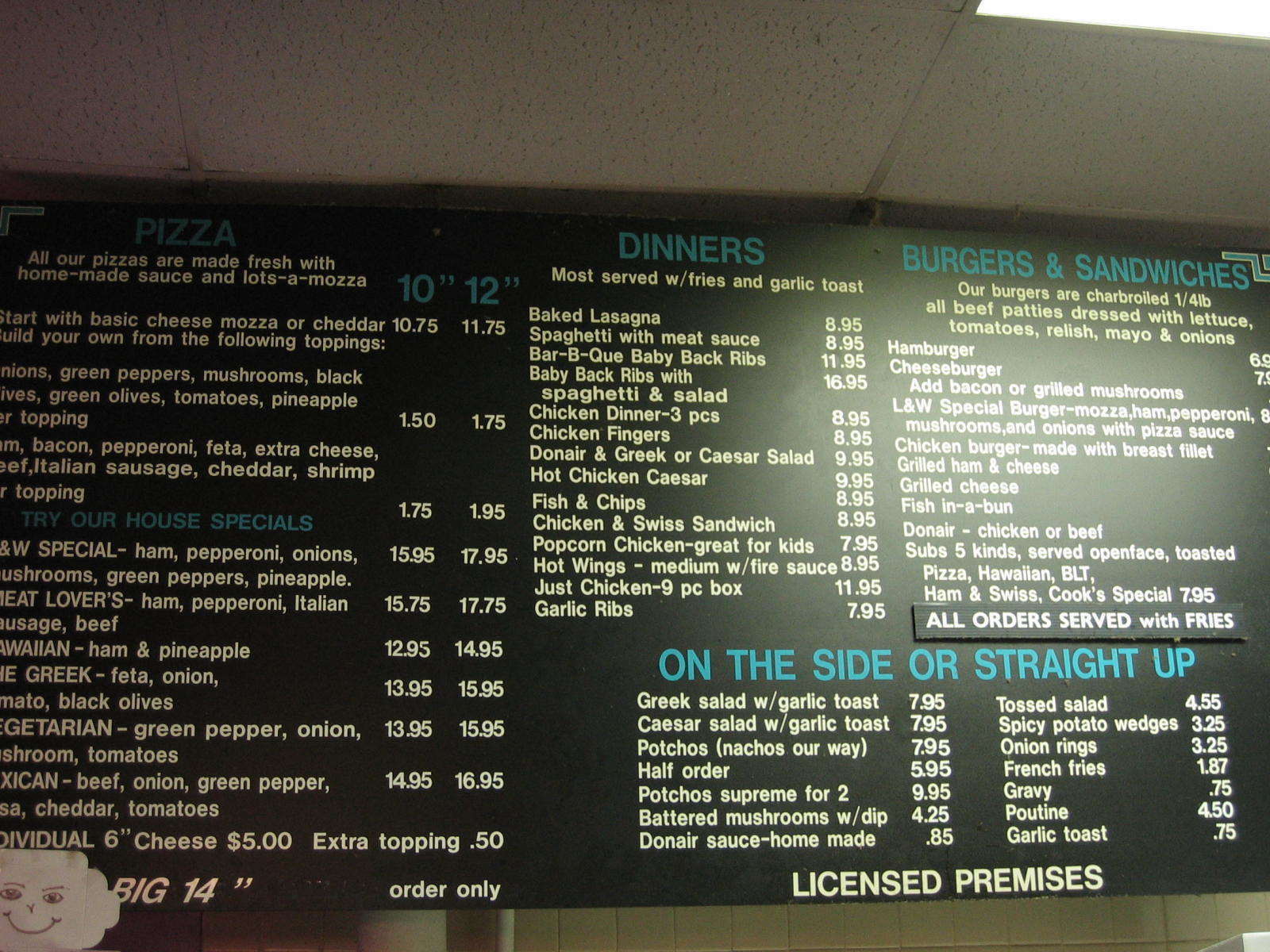This photograph captures a detailed view of a restaurant menu, giving an impression of an all-American, down-home cooking establishment specializing in meat-based dishes. The menu itself is black with white text for the items and striking giant blue text for the various sections.

In the top left corner of the menu, though the image is somewhat dark, the blue text section labeled "Pizza" is visible. Descriptions of the different pizzas can be partially read, though their names are obscured. Price comparisons for 10-inch and 12-inch pizzas are clearly displayed towards the top right section of the menu, where lighting is brighter, providing a clear view.

Moving towards the bottom left, there's a prominent section enticing customers to "Try Our House Special." While the names of the specials are not easily visible, their descriptions are partially legible, giving a sense of the offerings.

In the center of the menu at the top, there's a section labeled "Dinners," and on the bottom right, another section labeled "On the Side or Straight Up," likely listing side dishes and straightforward meal options.

Finally, the top right corner of the menu features a brightly lit section dedicated to "Burgers and Sandwiches," which outlines the sandwich options available at this all-American eatery.